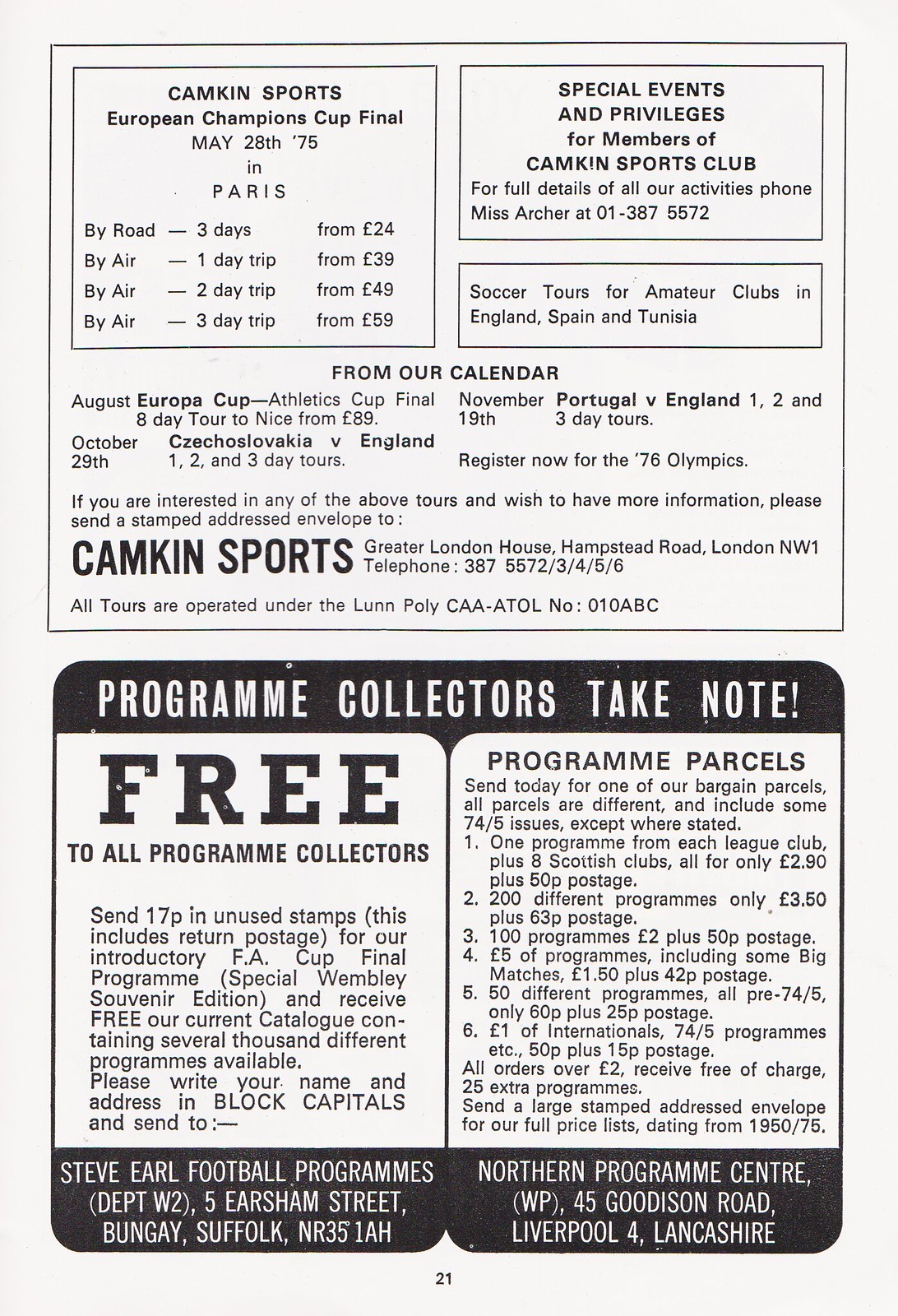This page, reminiscent of a magazine ad, is from Kamkin Sports, promoting the European Champions Cup Final held on May 28, 1976, in Paris. The clean, black-on-white print details travel packages and special events, specifically offering road trips starting at £24 for three days and various air travel options, ranging from one-day trips at £39 to three-day trips at £59.

The ad highlights exclusive events and privileges for Kamkin Sports Club members, featuring a variety of soccer tours for amateur clubs in England, Spain, and Tunisia. Interested parties are encouraged to contact Ms. Archer for more information at 01-387-5572 or send a stamped address envelope to Kamkin Sports in Greater London for a comprehensive list of activities.

Additional tours are also advertised from their calendar, including an 8-day tour to Nice for the August Europa Club Athletics Cup Final (£89), and various tours for international matches like Czechoslovakia vs. England on October 29, and Portugal vs. England on November 19.

For program collectors, the ad offers free introductory FA Cup Final Programs if 16 pence in unused stamps are sent. Detailed offers for program bundles are presented, including one program from each league club and eight Scottish clubs for £2.90 plus 50 pence postage, and parcels containing hundreds of different programs starting from £2.00 plus postage.

This promotional content, situated on page 21, underscores Kamkin Sports' extensive array of tours and collectibles, catering to devoted soccer enthusiasts and travelers alike.